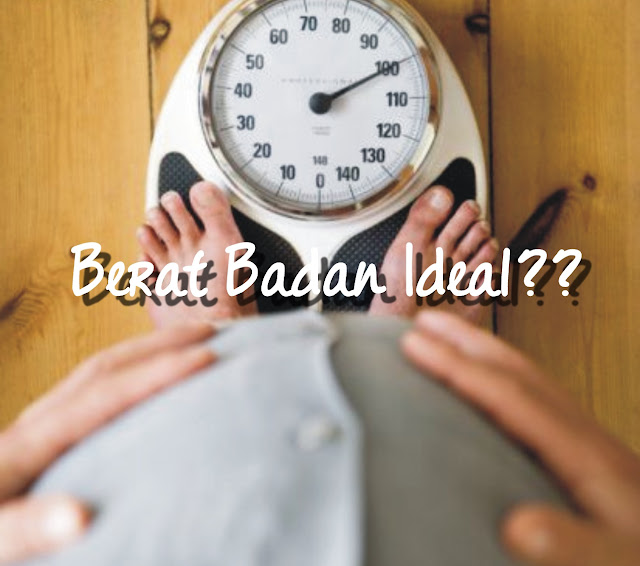A top-down image shows a person standing barefoot on a white bathroom scale with black textured grips for the feet. The scale, featuring a white face with a silver rim and a black dial, points to 190 on the upper right side. The person, whose hands rest on their midsection, wears a gray button-up shirt. The scale is placed on medium brown hardwood flooring. Across the center of the image, white text reads "BERAT BADAN" followed by "Ideal???" The feet and scale are in focus, while the person’s torso appears slightly blurred.